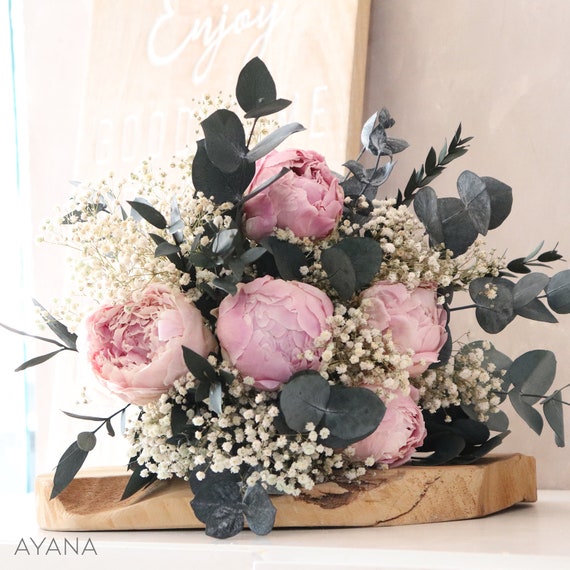Inside a softly lit room, a meticulously arranged artificial floral bouquet takes center stage. The bouquet features five large, pink flowers that resemble peonies or possibly primroses, some of which are still in the early stages of blooming. Interspersed among the pink flowers are sprigs of delicate baby's breath and dark gray eucalyptus leaves, contributing to the lush arrangement. The bouquet is set on a rustic, unfinished wooden slab, which rests on a white table or countertop. A wooden sign behind the bouquet bears the word "ENJOY" in white script, though the additional wording beneath is obscured by bright lighting. The background includes a pink-gray wall and a finished piece of wood in grays and whites, accentuating the rustic charm. The lower left corner of the image is marked with the name "AYANA," suggesting the possibility of the image being used as a greeting card or attributed to the creator of the arrangement.